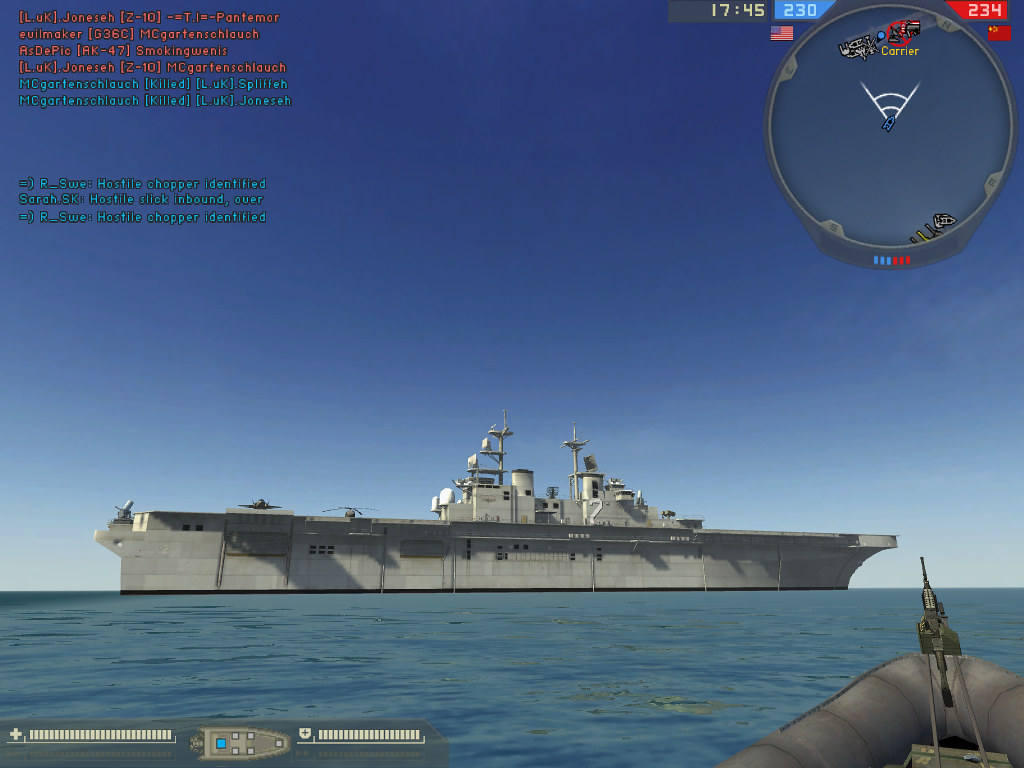A detailed screenshot from a highly realistic 3D video game or simulator. The image showcases an ocean setting under a clear blue sky. Dominating the scene is a large, gray aircraft carrier with a helicopter or fighter jet on its deck, and a building equipped with multiple radar units. The player's perspective is from a small inflatable boat equipped with a gun, visible in the lower right corner of the screen. 

In the upper right-hand corner, a mini-map is displayed showing the player's boat as a small blue icon moving towards the aircraft carrier, which is labeled "carrier" in yellow. The map also features a radar-like white overlay indicating the player's facing direction.

In the upper left-hand corner, a text chat reveals player interactions in red and blue letters, featuring names like Jonesy, Pontymore, The Evil Maker, 336C, McGardenshlock, and others. It includes in-game messages such as "McGardenshlock killed Spilfa" and "hostile chopper identified."

At the bottom left, a health bar with a heart symbol and ticks indicates the player's health status, accompanied by what seems to be an armor bar. Both bars use white tick marks on a sliding scale format.